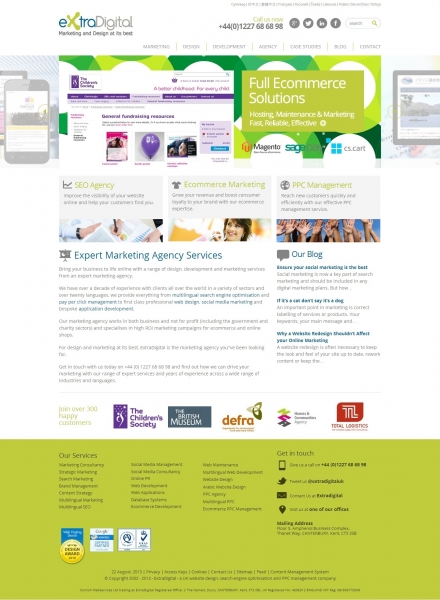This is a detailed screenshot of the "Extra Digital Marketing and Design" website, showcasing the company's comprehensive marketing and design services. The text is mostly small and blurry, making it difficult to read, but the site's purpose is evident. At the top, there's a UK phone number prompting visitors to call, and gray social media icons for Twitter, LinkedIn, and Facebook are aligned next to a search bar.

Below this section, there's a screenshot of another website, likely an example of Extra Digital's work. Faded in the background are additional screenshots of phones and tablets, suggesting a mini-portfolio of the company's projects. A prominent green text box highlights their offerings: "Full E-commerce Solutions, Hosting, Maintenance, and Marketing, Fast, Reliable, and Effective," accompanied by green circular graphics.

Further down, there's a detailed list of the company's services, emphasizing their expertise as an SEO agency, e-commerce marketing, and PPC management provider. Various stock photos are scattered throughout, including images of someone filling out paperwork, a smiling woman, and raised hands, adding a personable touch. On the right side, there’s a section titled "Our Blog," though the accompanying text is illegible.

Logos of prominent clients, such as Children's Society, the British Museum, DFRA, and Total Logistics, are displayed, signifying the company's credibility. At the bottom, there's a site map with various links, facilitating navigation throughout the website.